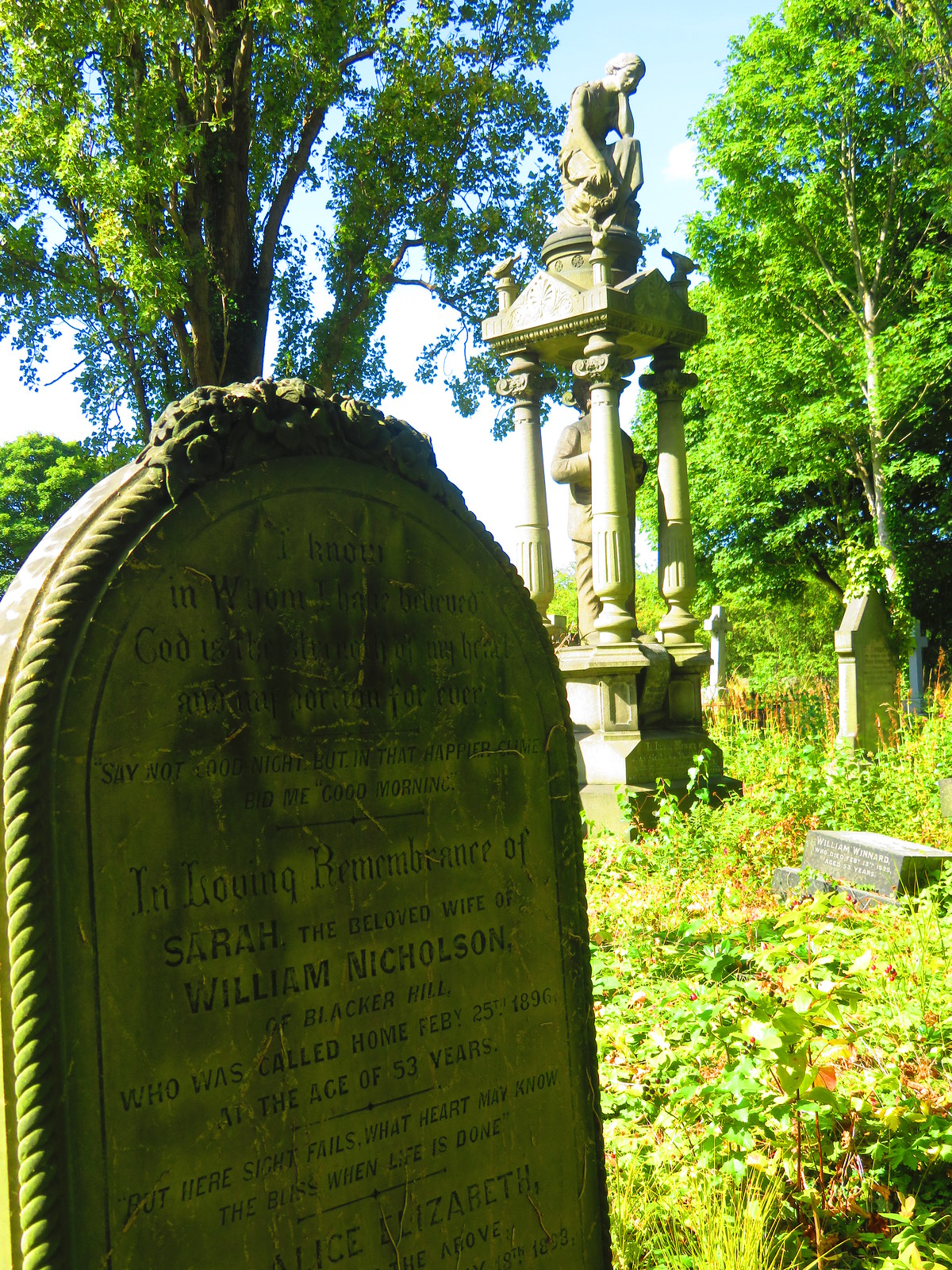On a clear and sunny day with blue skies adorned with a few clouds, the image captures an old cemetery surrounded by lush, green deciduous trees that cast sporadic shadows on the ground. The somewhat overgrown foliage adds to the rustic charm of the scene. At the forefront stands a gravestone with an oval top and intricate edging, reading, "In loving remembrance of Sarah, the beloved wife of William Nicholson of Blacker Hill, who was called home February 25, 1896, at the age of 53 years. But here sight fails what heart may know, the bliss when life is done." Below this inscription, the name "Alice Elizabeth" is faintly visible.

In the background, various gravestones can be seen, including one resembling a cross and another rectangular-shaped stone on the ground. Dominating the scene is an impressive statue featuring a man with his head in his hand, perched atop four pillars with another figure standing among them. The cemetery, filled with intriguingly shaped headstones suggesting granite, exudes an air of historical significance and old-world serenity.